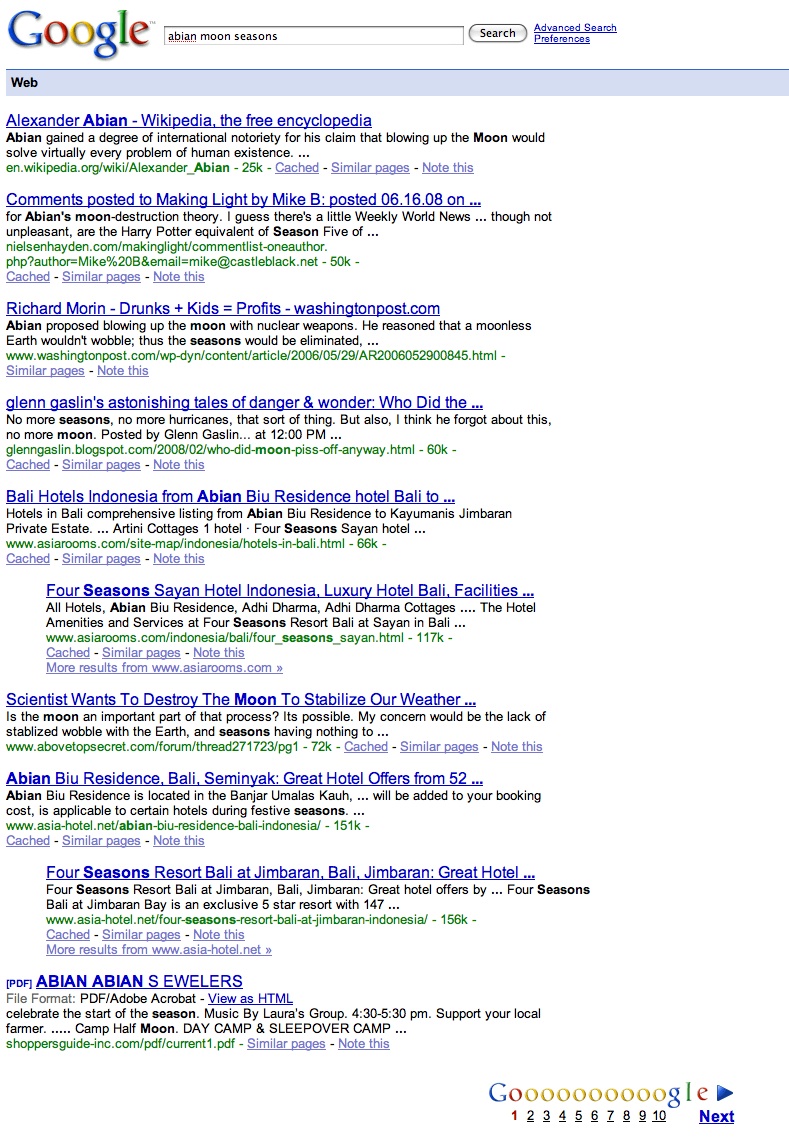**Caption:**

"This screenshot captures a browser window displaying search results for 'Abian moon seasons.' The first result links to Alexander Abian's Wikipedia page. The second result is a comment posted by Mike B on Making Light, timestamped 16:08. Following that is a link to an article by Richard Moran titled 'Drunks Plus Kids Equal Profits,' published by The Washington Post. Another result features 'Glenn Glassland's Astonishing Tales of Danger and Wonder,' with mention of Bali Hotels in Indonesia and the Abian Blue Residence Hotel in Bali. Continuing down the list, the search results include the 'Four Seasons Savian Hotel' in Indonesia, highlighting its luxury facilities in Bali. There is a result discussing scientists' desire to destroy the moon to stabilize Earth's weather, raising concerns about its impact on Earth's axial wobble. Additional entries reference the Abian Blue Residence in Seminyak, Bali, and the Four Seasons Resort in Jimbaran, Bali. The final results include Abian Jewelers, which appears unrelated to the initial query."